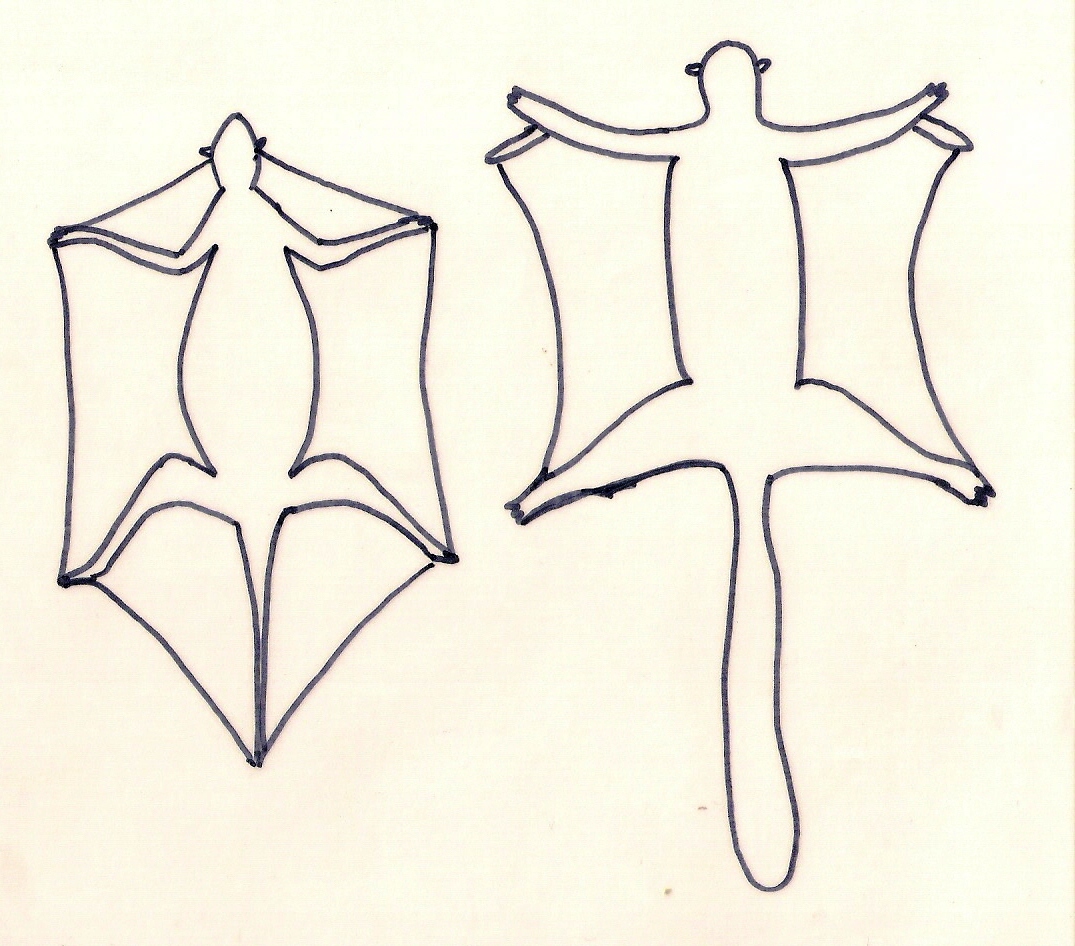The image depicts two minimalist black marker or pen sketches of flying squirrels on an ivory background. Both illustrations are top-down views of the animals with their limbs outstretched to display their gliding membranes. The left squirrel's webbing is more extensive and connects from its chin to its forepaws, from its forepaws to its back paws, and from its back paws to its tail, creating six sections of webbing. The right squirrel has a more conventional depiction, with the gliding skin stretching only between its forepaws and back paws, leaving its head and tail free. Neither sketch includes detailed facial features or fur, focusing instead on the outlines and basic body structure to emphasize the gliding membranes.